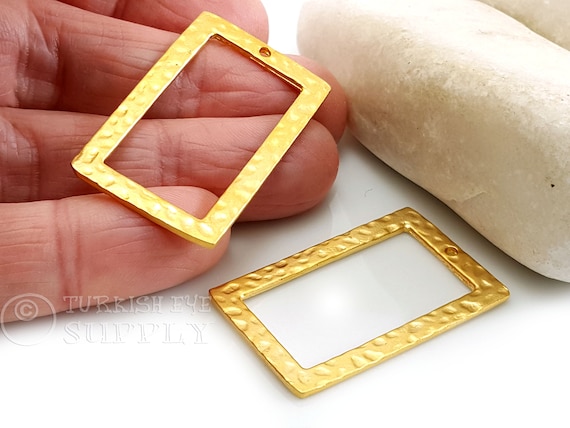This is a detailed photograph showcasing a pair of rectangular, gold-toned earrings, likely an advertisement for clay earrings by "Turkish Eye Supply," as indicated by the watermark. The image features a hand on the left side, holding one of these earrings, highlighting its hammered, frame-like design with an opening in the middle and a circular hole at the top for attachment. Near the hand, there is a second, identical earring resting flat on a white surface, possibly a fluffy pillow. The earrings appear to be about the length of a pinky finger and have a metal finish, suggesting they could be made of gold or a gold-like material.